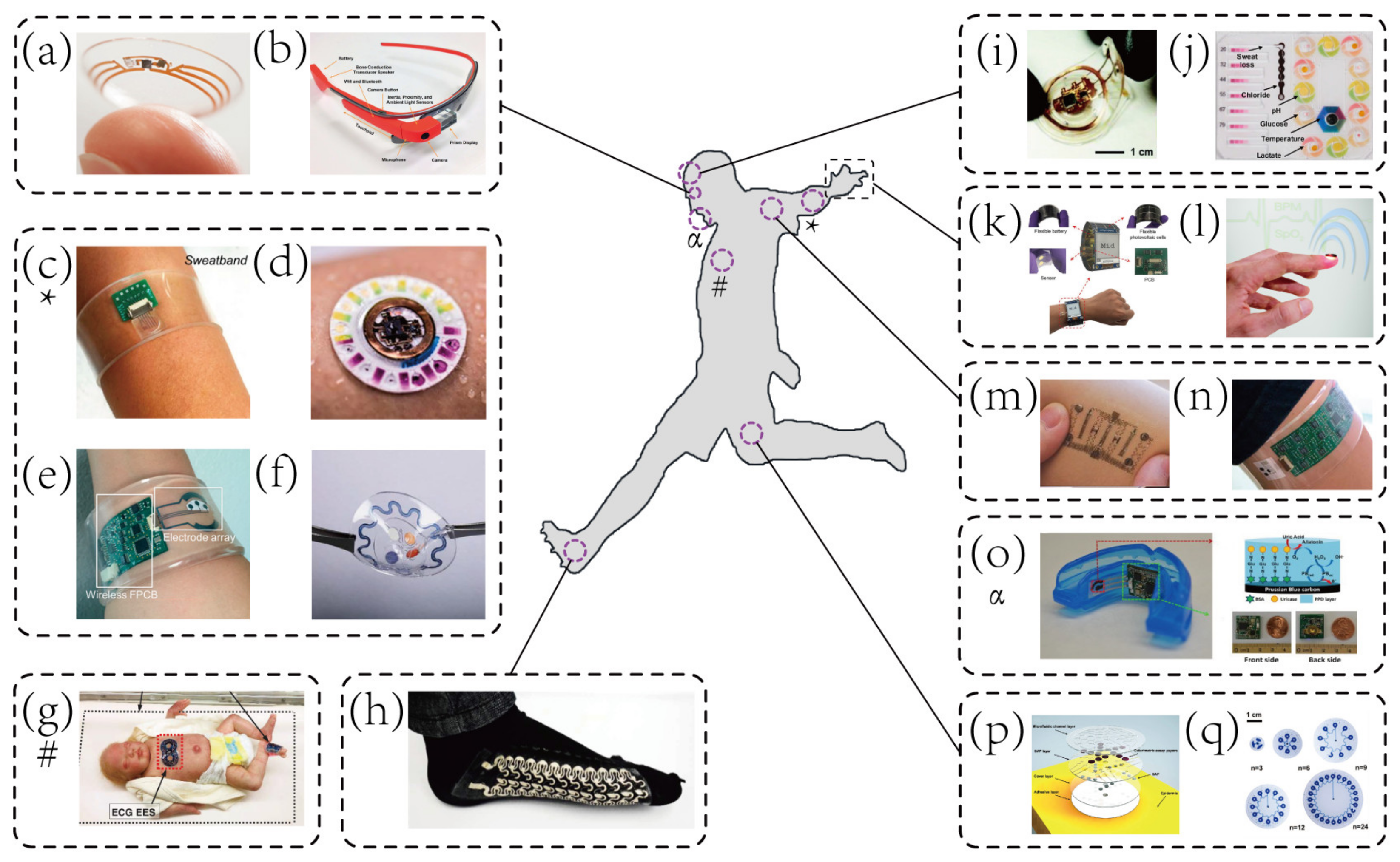The image is a detailed diagram featuring a gray silhouette of a human figure in a dynamic running or jumping stance, with one leg pointing downwards to the left and the other bent at the knee pointing towards the middle right. The figure's outstretched arms extend behind it. Surrounding the silhouette are various concentric circles positioned on different parts of the body, each connected by blue lines to a series of labeled sidebars situated to the left and right of the figure.

On the left side, the sidebars are organized into boxes with dotted or dashed black lines, containing letters A to H, each accompanied by images of different pieces of equipment. Specifically, Box A includes an unspecified item, Box B features special glasses with attached paraphernalia that could be a camera or light, and Box H appears to show a special pair of socks.

To the right, the boxes are labeled I to Q, similarly containing images of diverse items. Box O, for instance, displays a blue mouth guard intended for dental protection. These boxes collectively depict various pieces of equipment associated with the different body parts circled in the main figure.

Overall, the detailed diagram provides a comprehensive visual inventory of equipment, categorized and linked to specific body regions via letters and images, encapsulating an intricate system designed for a specialized purpose, possibly related to athletic or medical applications.